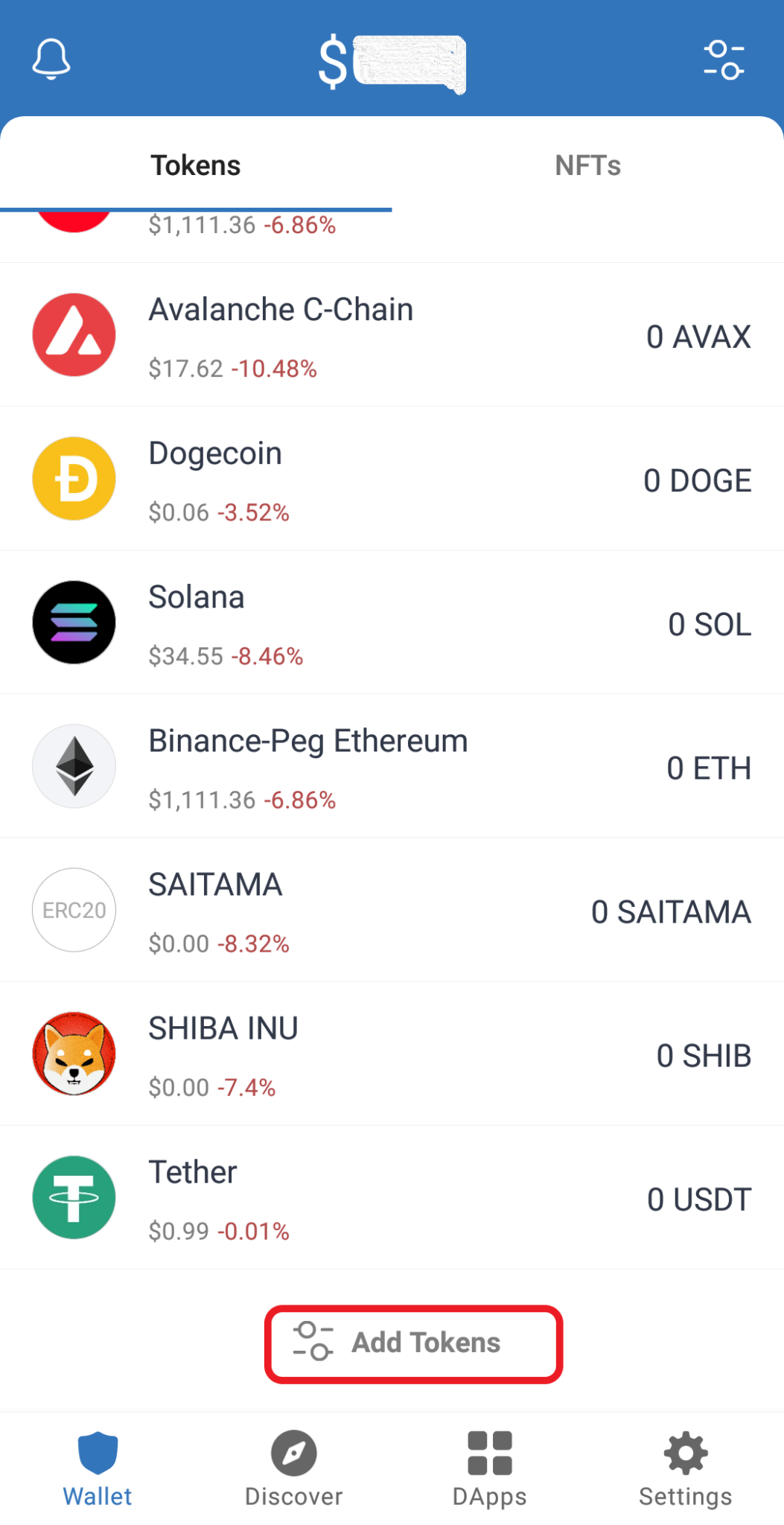**Detailed Caption for Image:**

The image is a screenshot depicting various cryptocurrency denominations. The top section features a blue bar containing a bell icon on the left. On the right side of this bar, there are two parallel lines, each ending in a circle. Centrally located in this bar is a dollar sign accompanied by a text box icon. Below this bar, there are two categories labeled "Tokens" and "NFTs," with the "Tokens" category highlighted. 

In the "Tokens" category, the following details are listed:

1. An unidentified token (name and icon not visible) showing only a dollar amount and a percentage change.
  
2. Avalanche (AVAX), indicated by a red circle with a white triangle and a line through it. It reads "Avalanche C-Chain" with a value of $17.62, showing a decline of 10.48%, and zero AVAX.

3. Dogecoin (DOGE), marked by a yellow dot with a white "D" and a line through the left side of the "D." It reads "Dogecoin," spelled out as D-O-G-E-C-O-I-N, with a value of $0.06, down by 3.52%, and zero DOGE.

4. Solana (SOL), displayed with its respective icon, and listed at $34.55, down by 8.46%, and zero SOL.

5. Binance-Peg Ethereum (ETH), written as E-T-H-E-R-E-U-M, valued at $1,111.36, down by 6.86%, and zero ETH.

6. Saitama (SAITAMA), with its icon and listed value of $0.00, down by 8.32%, and zero SAITAMA.

7. Shiba Inu (SHIB), denoted by a fox within a red circle. It reads "Shiba Inu," spelled out as S-H-I-B-A I-N-U, with a value of $0.00, and zero SHIB.

8. Tether (USDT), with its value listed at $0.99, down by 0.01%, and zero USDT.

At the bottom of the list is a highlighted tab labeled "Add Tokens," outlined in red. Additionally, there are four navigation icons across the bottom: Wallet, Discover, D-Apps, and Settings.